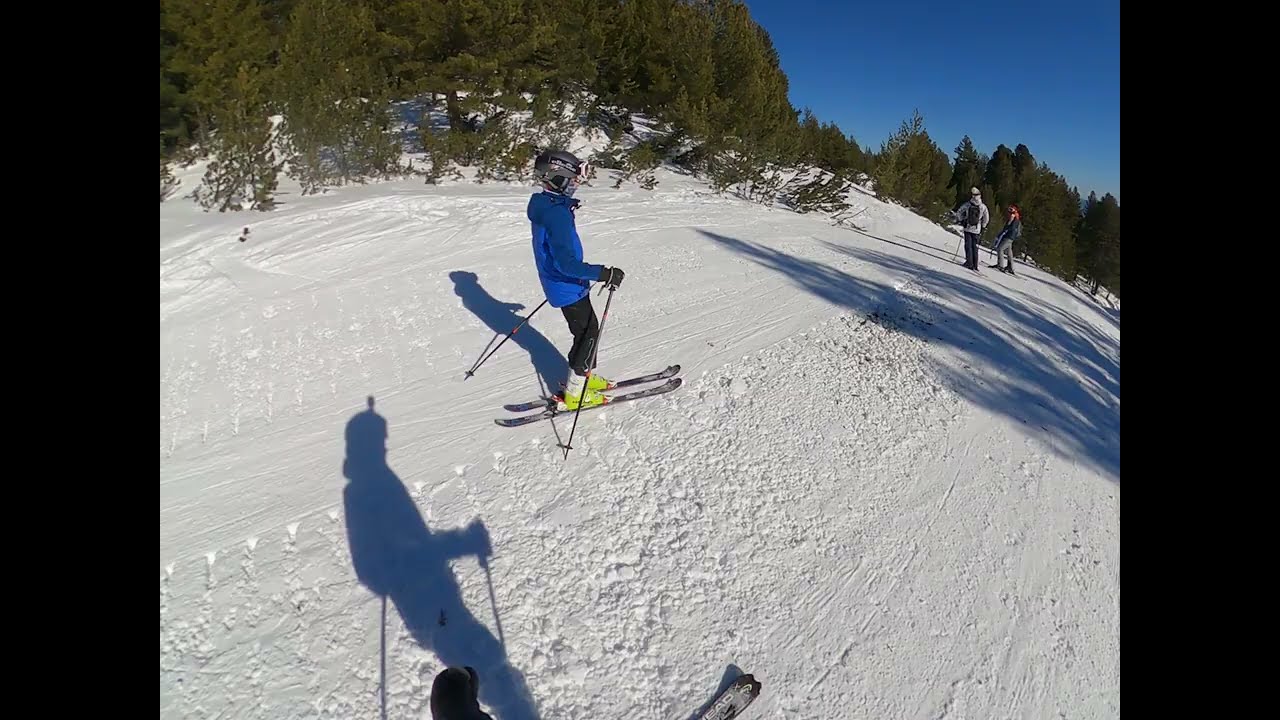A detailed daytime photograph capturing a vibrant ski scene on a snow-covered mountain. The image centers around four skiers with a backdrop of a clear, blue sky and numerous evergreen trees. Prominently in the foreground, a skier in a blue jacket, black gloves, black pants, green ski boots, and a helmet stands confidently with ski poles in hand, casting a distinct shadow on the smooth, freshly curated snow. Off to the side, only the shadow of another person is visible, indicating their presence without showing their form. In the distance, two additional skiers can be seen, one of them a man wearing a gray shirt and carrying a black backpack, and the other a woman with red hair. Both are equipped with ski poles and are positioned against the snowy, unblemished terrain. The entire scene is bathed in bright sunlight, highlighting the serene beauty of the outdoor winter setting.